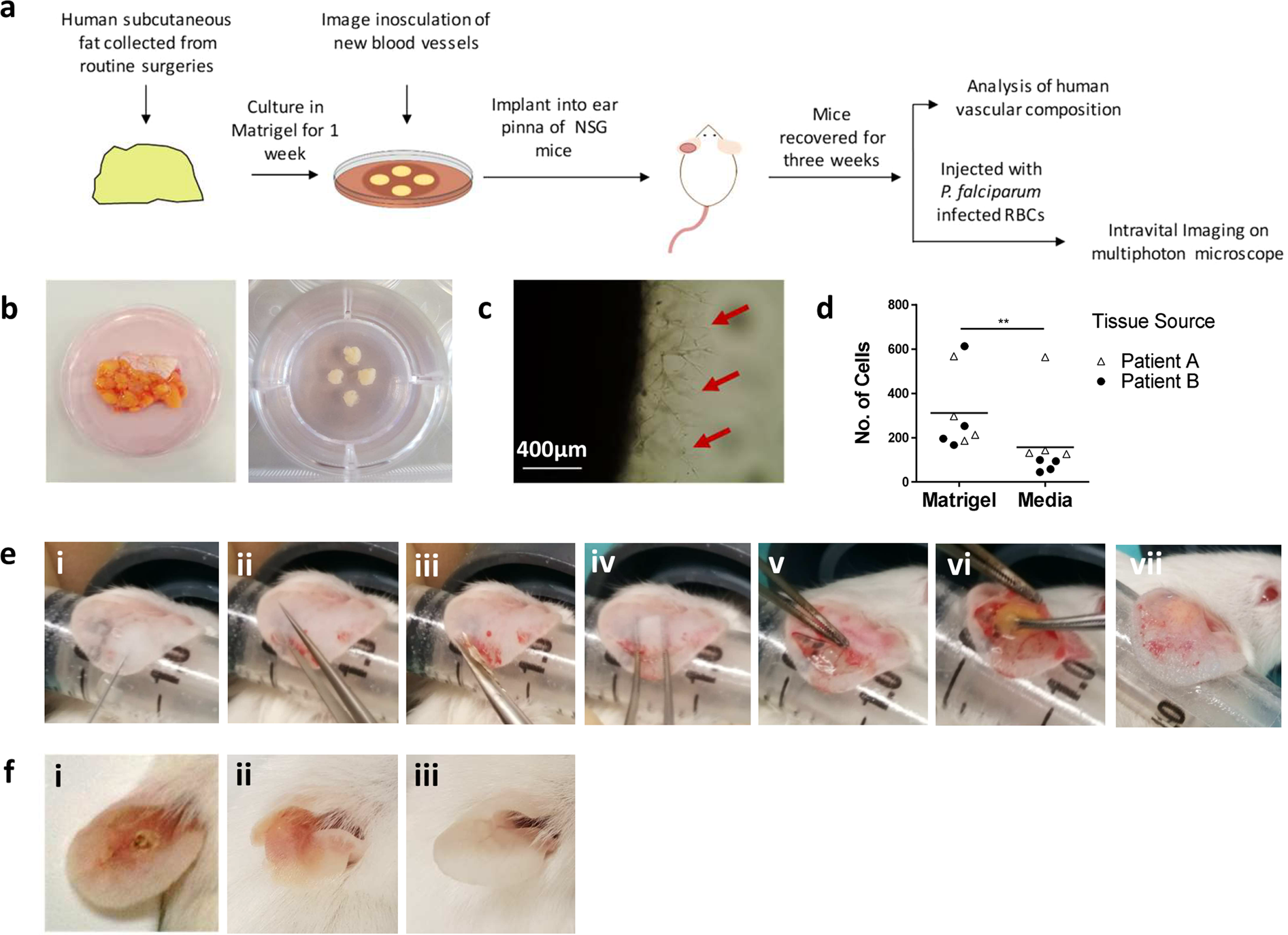The image depicts a detailed scientific procedure involving human subcutaneous fat collected from routine surgeries. The fat is cultured with matrigel for one week, leading to the inosculation of new blood vessels. These cultured tissues are then implanted into the ear pinna of NSG mice. The mice are allowed to recover for three weeks before analysis. The procedure is thoroughly illustrated through several rows of images labeled A through F. Row A details the initial collection and culture of human fat, while the following rows (B to E) depict the stages of implantation, recovery, and various analyses including intravital imaging using a multi-photon microscope. Specifically, row B shows close-ups of human skin with fat and the tissue source, while row F includes images before and after an ulcer removal, illustrating the changes in tissue post-implantation. The ultimate goal appears to be observing the impact of injecting falciparum-infected red blood cells into the mice, with emphasis on the development of new blood vessels and vascular composition.